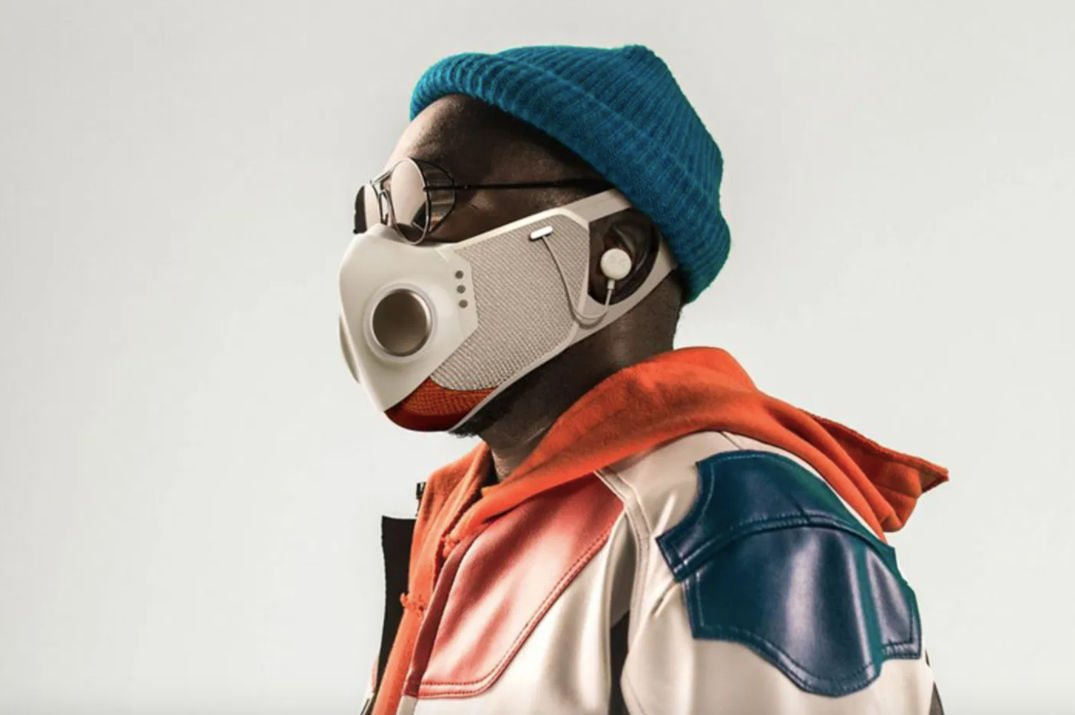This is a detailed profile view of an African-American man against a white background, showcasing a high-tech appearance ready for winter activities. He wears circular sunglasses and a high-tech face mask that is beige, red, and white with integrated earbuds. The earbuds connect to the mask by hooking towards the front cheek area. The mask features silver breathing filters and sits just above a meticulously groomed beard visible at the top of his neck. He sports a blue knitted skull cap rolled up slightly to expose his forehead. His layered clothing consists of a striking red, white, and blue leather jacket with an orange hoodie underneath. The jacket features blue patches on the shoulders and red patches around the buttons, and the orange hoodie contrasts vividly, adding to his vibrant and tech-savvy winter look.